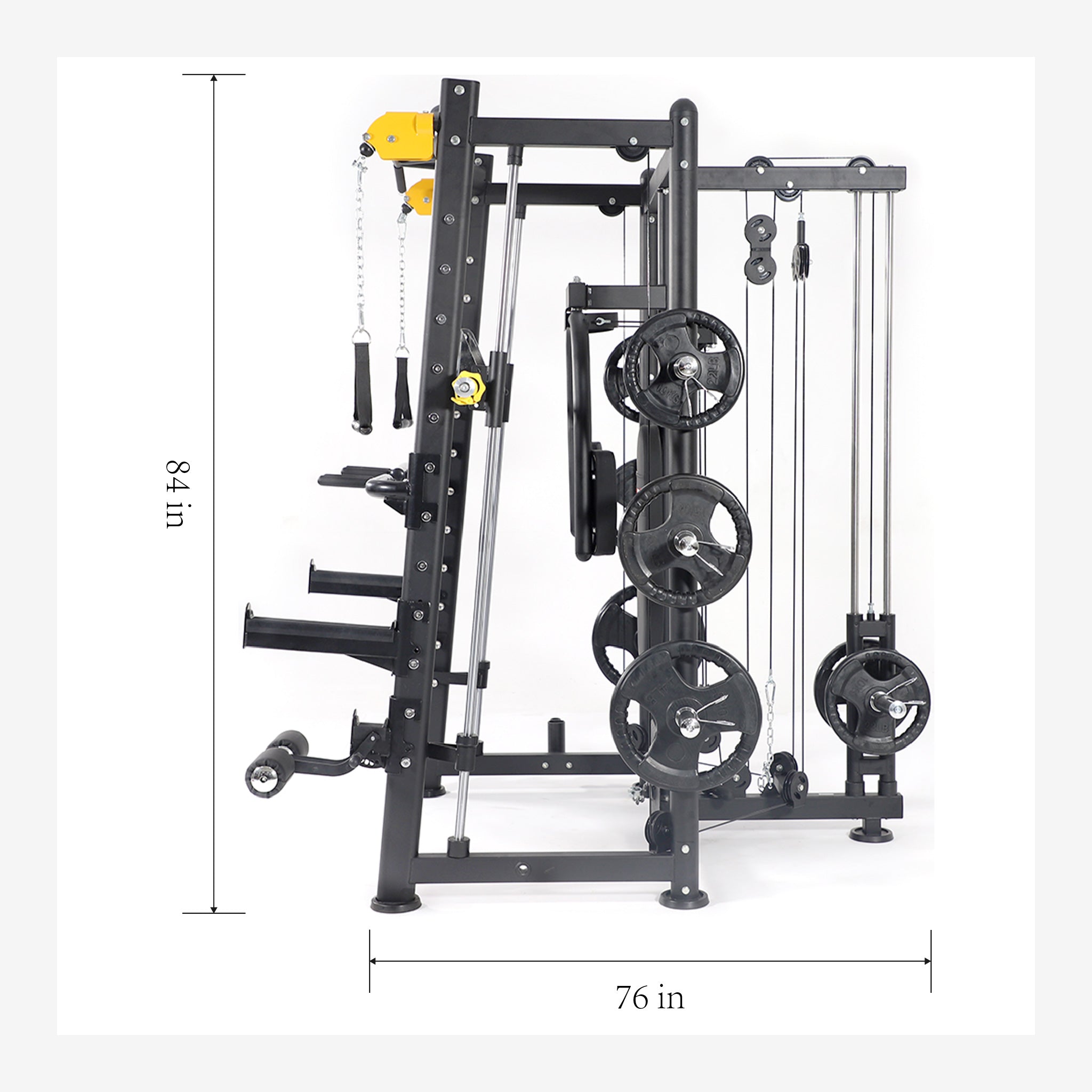The image features a side-view photograph of a large, complex piece of exercise equipment, set against a gray background within a white rectangle. The apparatus is mostly constructed from black metal, interspersed with several silver bolts and connecting pins, and a few yellow-painted components. On the left side, there are handles attached to strings, which appear to be part of a pulley or weight-lifting system. Above these handles are smaller grips, and straps are visible, indicating multiple points of resistance. 

White chains connect these straps to a yellow metal piece, adding to the intricate network of pulleys and cables visible throughout the machine. To the right, the equipment features bars that extend outward and then down, flanked by wheels on the outer sides. Additional strings and pulleys are located towards the bottom section. Measuring bars within the image indicate that the equipment stands 84 inches tall and spans 76 inches in width. This highly detailed and mechanical apparatus, with its assorted grips, wheels, and pulleys, suggests a multifaceted exercise machine designed to accommodate various forms of physical training, although its exact function may not be immediately recognizable from this angle.